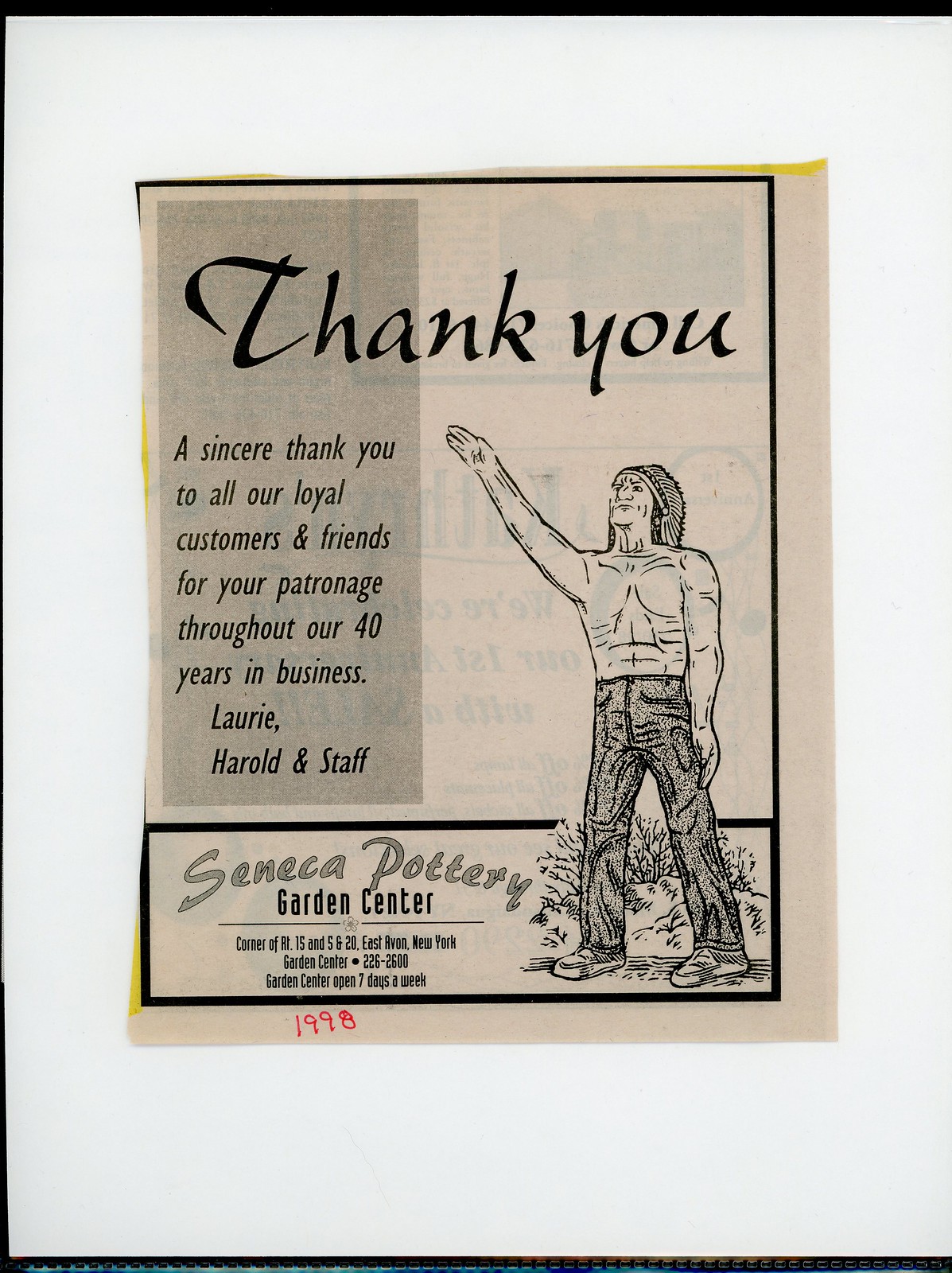The image is a photograph of an old, thin newspaper clipping with an off-white, aged appearance. You can faintly see text from the other side of the paper. The clipping is potentially framed, with a white matte and a thin black frame visible at the edges. At the top of the page, in cursive black font, it says "Thank you." To the left, within a light gray bar, the text reads: "A sincere thank you to our loyal customers and friends for your patronage throughout our 40 years in business, Lori, Harold, and staff." The central image features a shirtless Native American man, wearing a headdress, raising his right arm and gazing towards the left. At the bottom of the clipping, in a black rectangular box with offset text, it says, "Seneca Pottery Garden Center, corner of Route 15 and 5 and 20, East Haven, New York, Garden Center opens 7 days a week." In red ink, someone has written "1998." The text also includes a phone number, "226-2600."